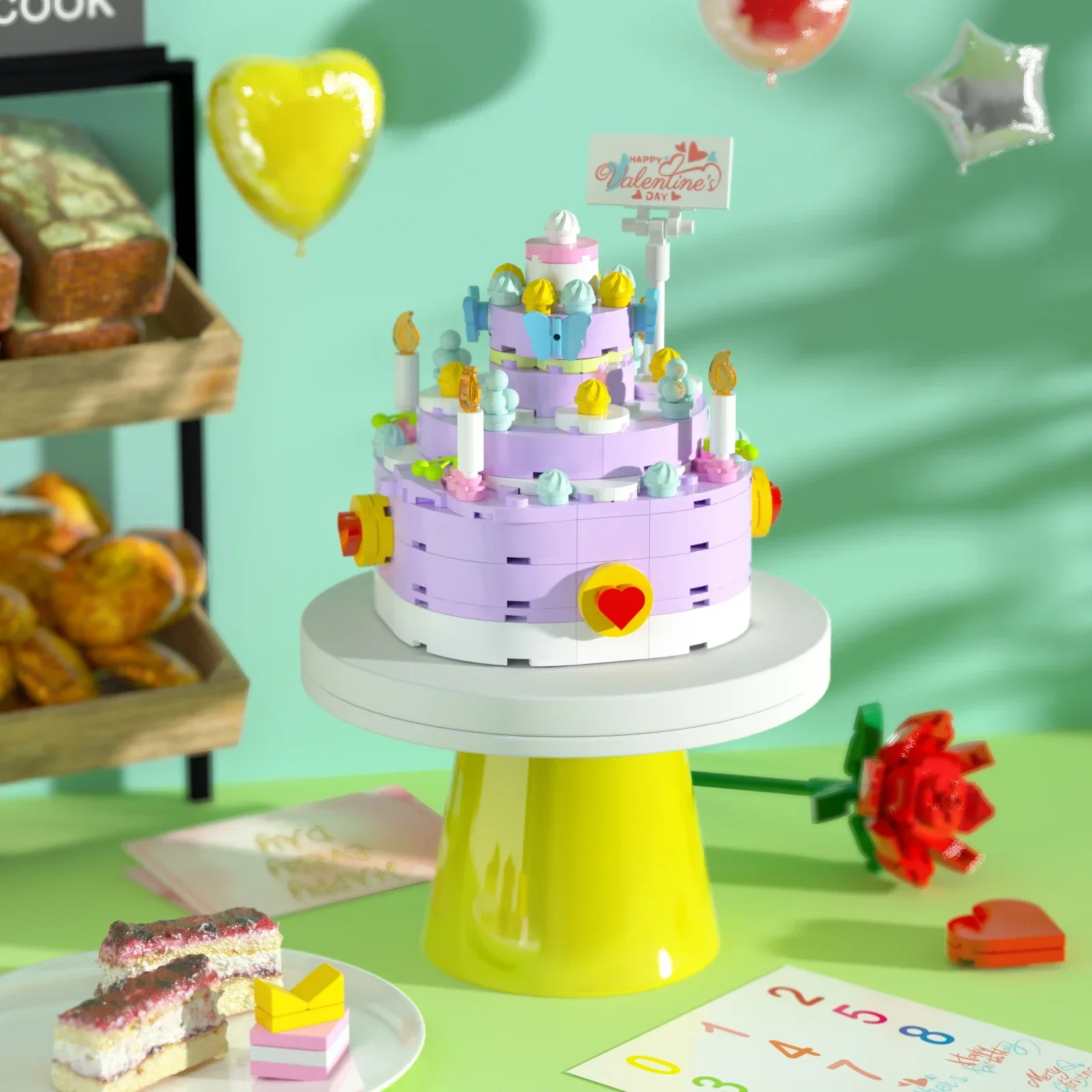The photograph features a vibrant, intricate display centered around what appears to be a light purple cake constructed entirely out of Lego-like plastic blocks, complete with large candles featuring yellow flames. The cake is adorned with a sign that reads "Happy Valentine's Day," decorated with small hearts. This cake sits on a yellow pedestal placed on a lime green table. In addition, there is a plastic rose positioned on the table beside the cake, and nearby, a white plate holds smaller plastic cakes and a tiny present with a bow, also seemingly made from Lego pieces. The backdrop includes mylar balloons and a small shelf stocked with assorted pastries and bread items. The overall theme suggests a celebration, possibly blending both birthday and Valentine's Day elements, as indicated by the romantic decorations and various baked goods displayed in a bakery-like setting.